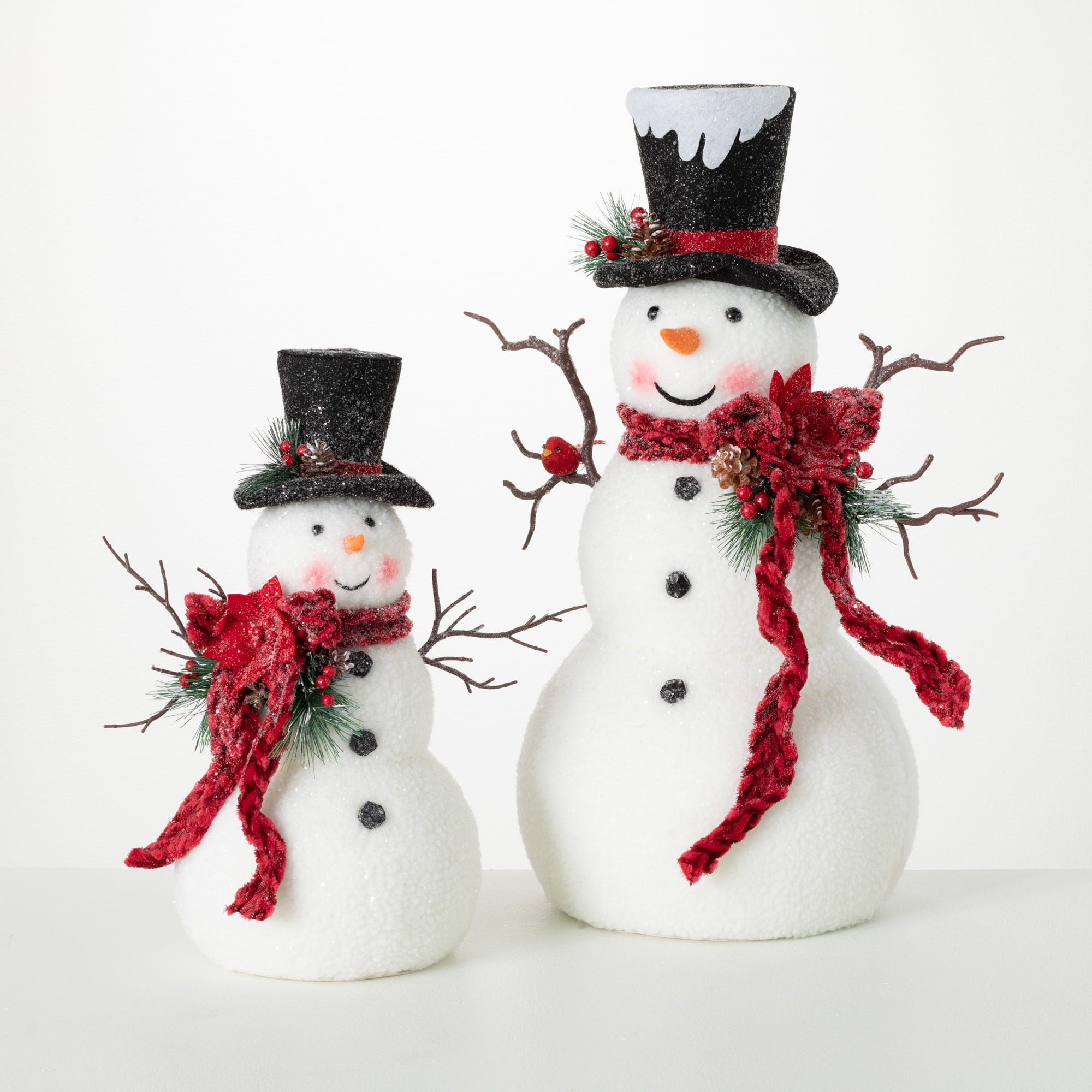This close-up photograph captures two charming snowman decorations crafted from a glistening, styrofoam-like material. The tableau features a larger "parent" snowman and a smaller "child" snowman, positioned side by side on a white table with a white backdrop, creating a cozy holiday scene. Both snowmen are constructed from three white, glittering spheres that decrease in size from bottom to top, mimicking traditional snowballs.

Each snowman is adorned with a black top hat featuring a red ribbon accented with festive holly, pinecones, and berries. The hats glisten subtly with a light sheen of glitter, and the larger snowman's hat also sports a charming cutout to represent a snowcap. Their cheerful faces are complete with two black eyes, a carrot nose, rosy cheeks, and a gentle smile.

They are wrapped in matching red scarves that include more of the decorative holly, pinecones, and berries. Tree branch arms extend from their sides, adding a natural touch to their whimsical appearance. Each snowman is detailed with three coal-like buttons down their front, enhancing their classic snowman look. A notable detail is the little red bird nestled under the arm of the larger snowman, adding an extra layer of warmth and charm to this delightful holiday scene.